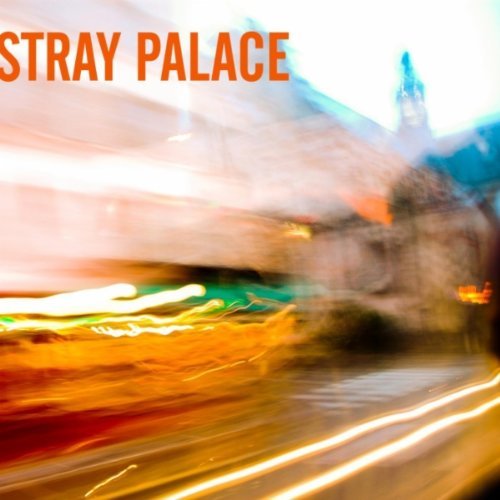This image captures a dynamic, time-lapse scene of a bustling street filled with streaks of light from passing cars, painting an almost impressionistic blend of colors including oranges, greens, reds, yellows, and whites. The overall atmosphere is quite blurry, suggesting motion, possibly taken from a moving vehicle. In the background on the top right, you can discern a faintly visible, blue-roofed building or steeple, adding to the urban landscape. The most clear and static element in this motion-filled image is the bold, orange text "Stray Palace" positioned in the top left corner, anchoring the otherwise fluid and abstract composition.